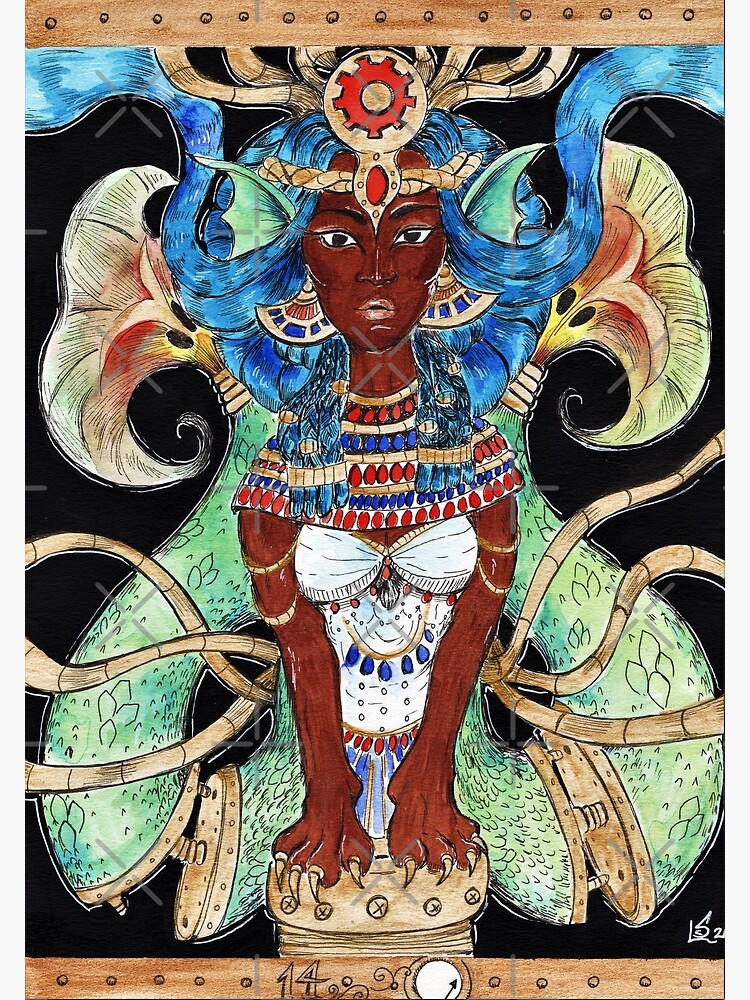The image is a contemporary art painting on a black background, featuring an African-American female figure adorned in mythological and possibly Egyptian-like decorations. She sits at the center of the painting, seated on a gold perch. Her outfit is a pristine white dress, complemented by an elaborate white neck piece that covers her shoulders. Her striking blue hair is styled in a Medusa-like manner, flowing behind her with the appearance of tentacles that have a greenish tinge originating from her lower back. The woman gazes straight ahead, and a subtle blue and gold necklace or ornament decorates her chest.

Adding to the mystique, she possesses paws with gold claws instead of hands. She wears a golden crown and matching golden earrings, while her broad necklace is adorned with red and blue dots. Reptilian-like ears peek through her blue tresses, enhancing her otherworldly appearance. On either side of her, what looks like a dragon's tail can be seen, further extending the mythological theme.

The painting is framed by a light golden brown border on the top and bottom, featuring small circular designs reminiscent of tacks. At the bottom, the number "14" is visible alongside a scroll design and a round white circle with an arrow through it. The artist's signature, resembling a symbol rather than a traditional name, is located in the bottom left-hand corner. The overall composition is vivid and colorful, blending elements from multiple mythological references.